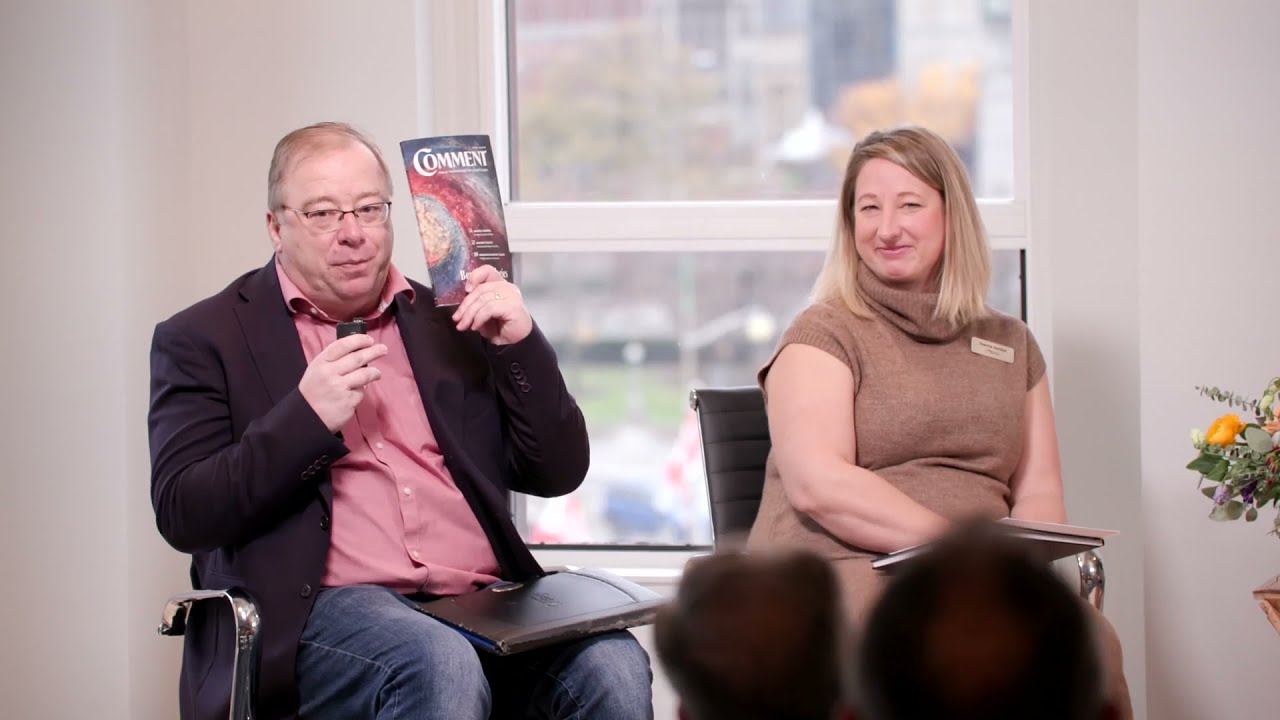This detailed image depicts a man and a woman seated next to each other, likely participating in a public talk or a meeting in an office setting. They are positioned in front of a window overlooking a sunny park, indicating they might be on a higher floor, such as the second or third story. 

The man, appearing to be in his 50s, has balding, thinning gray hair and wears glasses. He is dressed in a black sports coat paired with a pink button-up shirt and blue jeans. In his left hand, he holds up a magazine titled "Comment," while his right hand grasps a microphone. His demeanor suggests he is addressing the audience in front of him, whose heads are partially visible and are focused on the speakers.

To his right is a woman who is smiling warmly at the crowd. She is likely in her 40s, with shoulder-length blonde hair. She is wearing a short-sleeved brown dress or possibly a shirt and a tan sweater. A badge, possibly displaying her name, is draped over her shoulder. A bouquet of flowers, partially visible, adds a touch of elegance to the space. 

The setting, enhanced by the natural light streaming in from the window behind them, combined with the attentive audience, underscores the formal yet inviting atmosphere of the event.